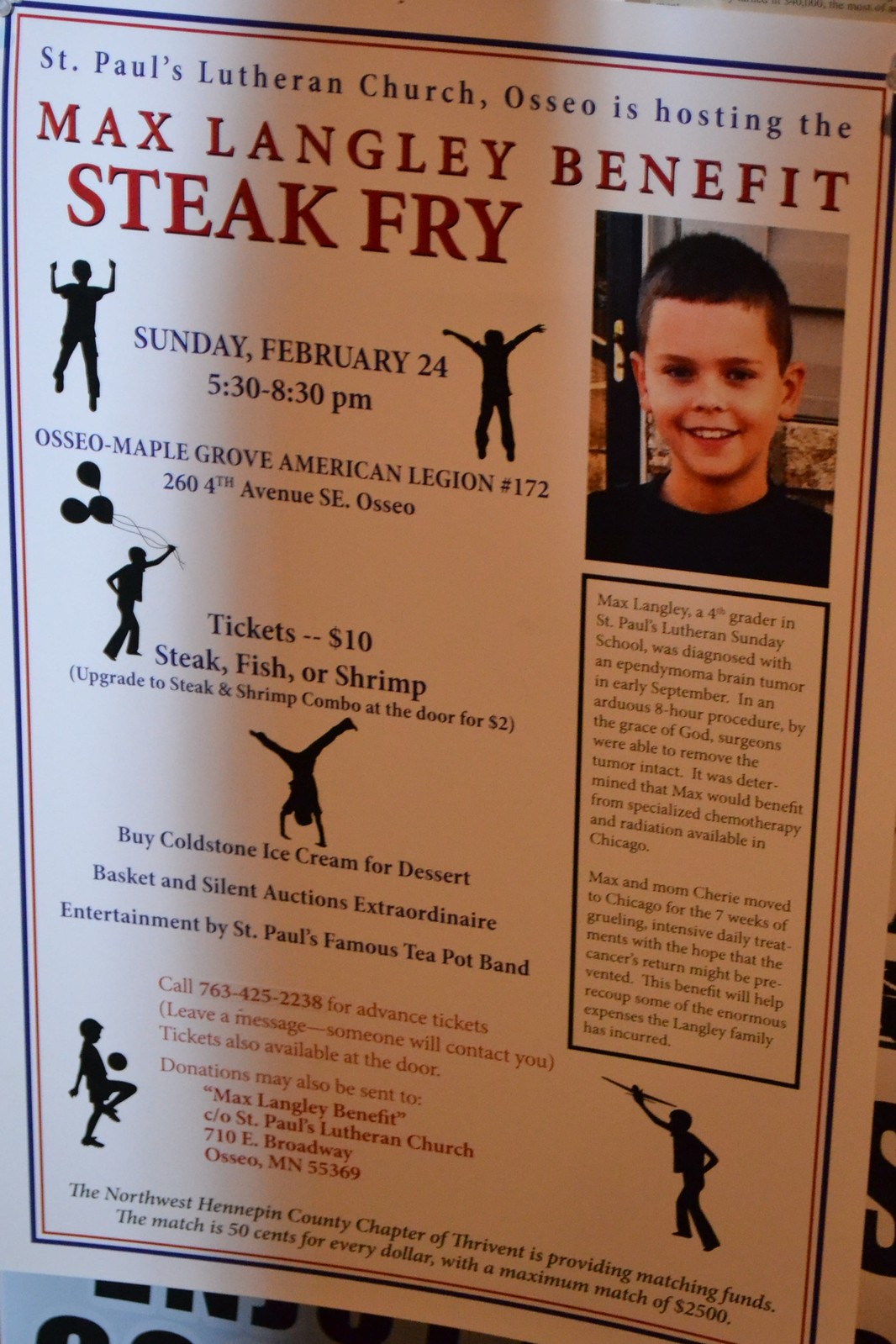The image is a detailed poster for a benefit steak dinner, designed to support Max Langley, a young boy with a brain tumor. At the top of the poster, written in blue, it states "St. Paul's Lutheran Church, Osseo is hosting the Max Langley Benefit Steak Fry." To the right side is a photo of Max Langley, estimated to be about eight or nine years old, smiling with short black hair and a black top, exuding a hopeful spirit.

To the left of his photo, there are two silhouette drawings of a boy; one with his hands above his head and another with arms outstretched. The event details, situated between these images, read, "Sunday, February 24, 5:30 to 8:30 p.m." Further below, there is another silhouette of a boy holding three balloons with details stating, "Osseo Maple Grove American Legion No. 172, 264th Avenue SE, Osseo."

The poster also includes additional elements like tickets information: "$10 for steak, fish, or shrimp. Upgrade to steak and shrimp combo at the door for $2." Some more silhouettes illustrate children in various playful poses, including a boy doing a handstand, another bouncing a ball, and one holding a model airplane. 

Highlighting the event, it is mentioned in blue writing that "Coldstone ice cream will be available for dessert," alongside a silent auction and extraordinary entertainment by "St. Paul's famous Teapot Band." The poster encourages people to call "763-425-2238" for advance tickets, though tickets are also available at the door. 

Lastly, at the bottom, there’s an option for donations to be sent to "Max Langley Benefit, care of St. Paul's Lutheran Church, 710 Broadway, Osseo, Minnesota 55369." Also mentioned is that the Northwest Hennepin County Chapter will provide matching funds of 50 cents for every dollar, up to $2,500.

This event is a communal effort to raise money to help cover medical expenses for Max Langley, encapsulated in a heartfelt and informative poster.